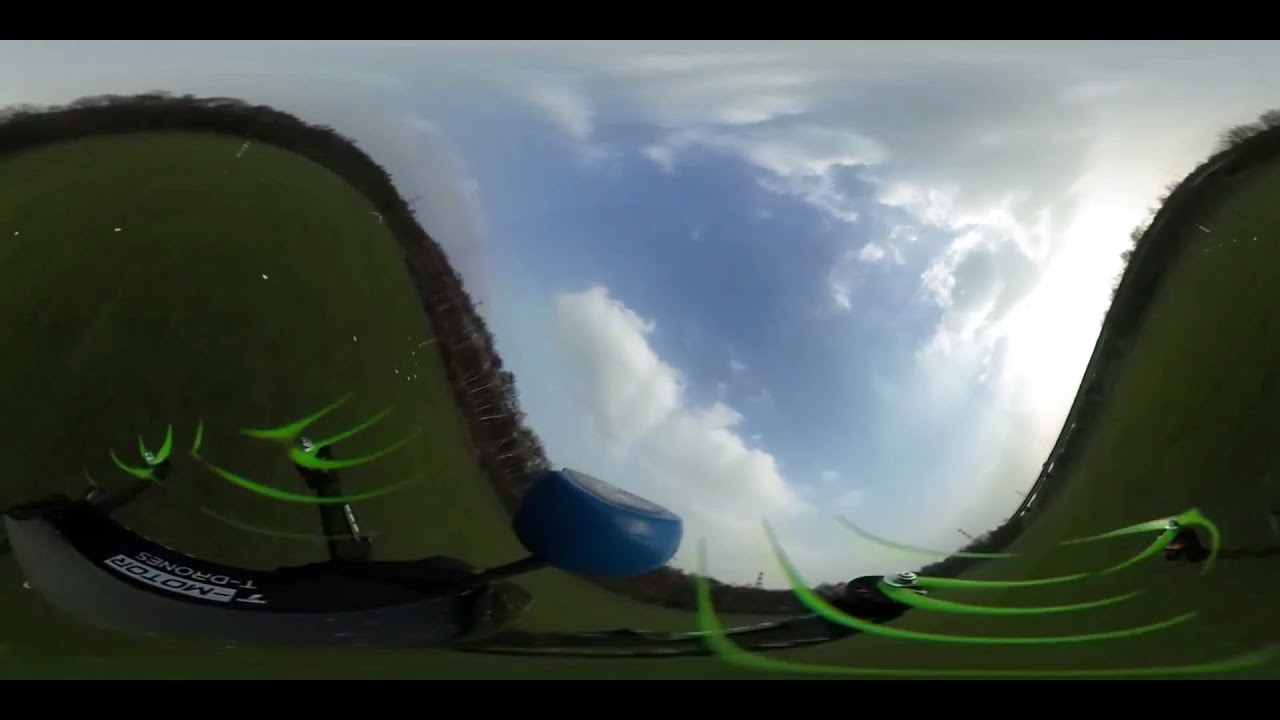In this fisheye panoramic photograph, a scenic outdoor view is captured, featuring a predominantly light blue sky interspersed with both gray and white clouds. Notably, the right side of the image reveals the sun subtly peeking through the clouds. The photograph presents a verdant, hilly landscape with an S-curve formed by two green hills sloping downward toward the center, topped with a line of trees bearing dark green leaves. A flat grass field extends across the bottom of the image, with a distinctive black drone in the foreground. The drone is equipped with propellers on its four corners and a bulbous blue camera projection jutting out from its front, marked with "T-motors" or "T-drones." The fisheye effect and the propellers give the picture a distorted look, creating a concave shape in the center. The photograph is clearly taken mid-flight, capturing the serene and expansive outdoor setting.